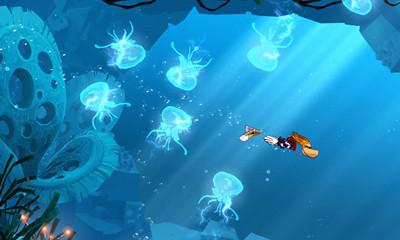This image portrays a computer-generated, underwater scene with a distinctive video game aesthetic, likely designed for mobile screens. The dreamy, predominantly blue landscape features various marine elements, including more than six ethereal, blue jellyfish dispersed across the scene, with a small red jellyfish appearing in the upper right. The setting includes a rocky outcrop extending from the top, along with vibrant underwater flora. On the left, glowing-tip plants and corals enhance the scene’s aquatic feel. The central right section of the image features a unique, limb-disconnected character who appears to be an iconic video game figure, potentially resembling a duck. This character is depicted swimming underwater with bubbles trailing behind. Additionally, there's a white, floating hand visible towards the middle, creating a mysterious and whimsical underwater adventure vibe. The interplay of light and detailed seabed vegetation, including a conspicuous gear-like plant structure with tentacle-like extensions, contributes to the overall immersive experience.